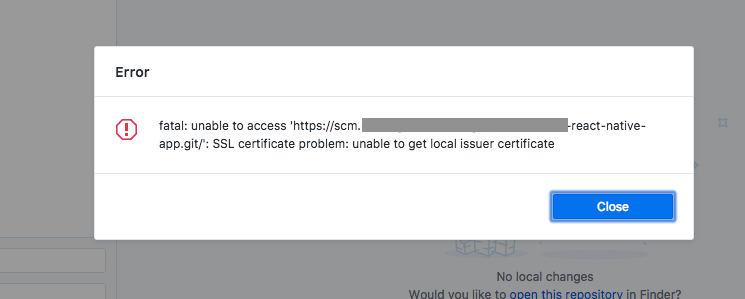The image displays an error message indicative of a technical issue encountered while accessing a web resource. The main body of the message is within a large, gray, rectangular box. Centrally positioned within this gray box is a smaller white box containing detailed text. 

In the upper left-hand corner of the white box, there is a red "error" label. Just below this label, an icon resembling a stop sign outlined in red with a red exclamation mark at its center signals the severity of the issue.

The main text starts with the word "Fatal:" emphasizing the critical nature of the error, followed by "Unable to access," implying a blockage in access. This is accompanied by a URL in HTTPS format, indicating a failed connection attempt to a repository likely located at "SCM..." (the remaining URL is grayed out and not fully visible).

The text continues, detailing a path structure: "slash react slash native slash." On the next line, there's a reference to a file path: "pp.git" followed by a backslash and more text detailing, "SSL certificate problem: unable to get local issuer certificate."

At the bottom of the white box, there is a blue button labeled "Close" in white text. Below this, in a faint gray area, a message reads, "No local changes. Would you like to open this repository in Finder?"

The overall depiction is a clear indication of an SSL certificate error preventing local access to a remote repository, complete with UI elements to interact with the notification, such as the option to close the message or further explore the repository.